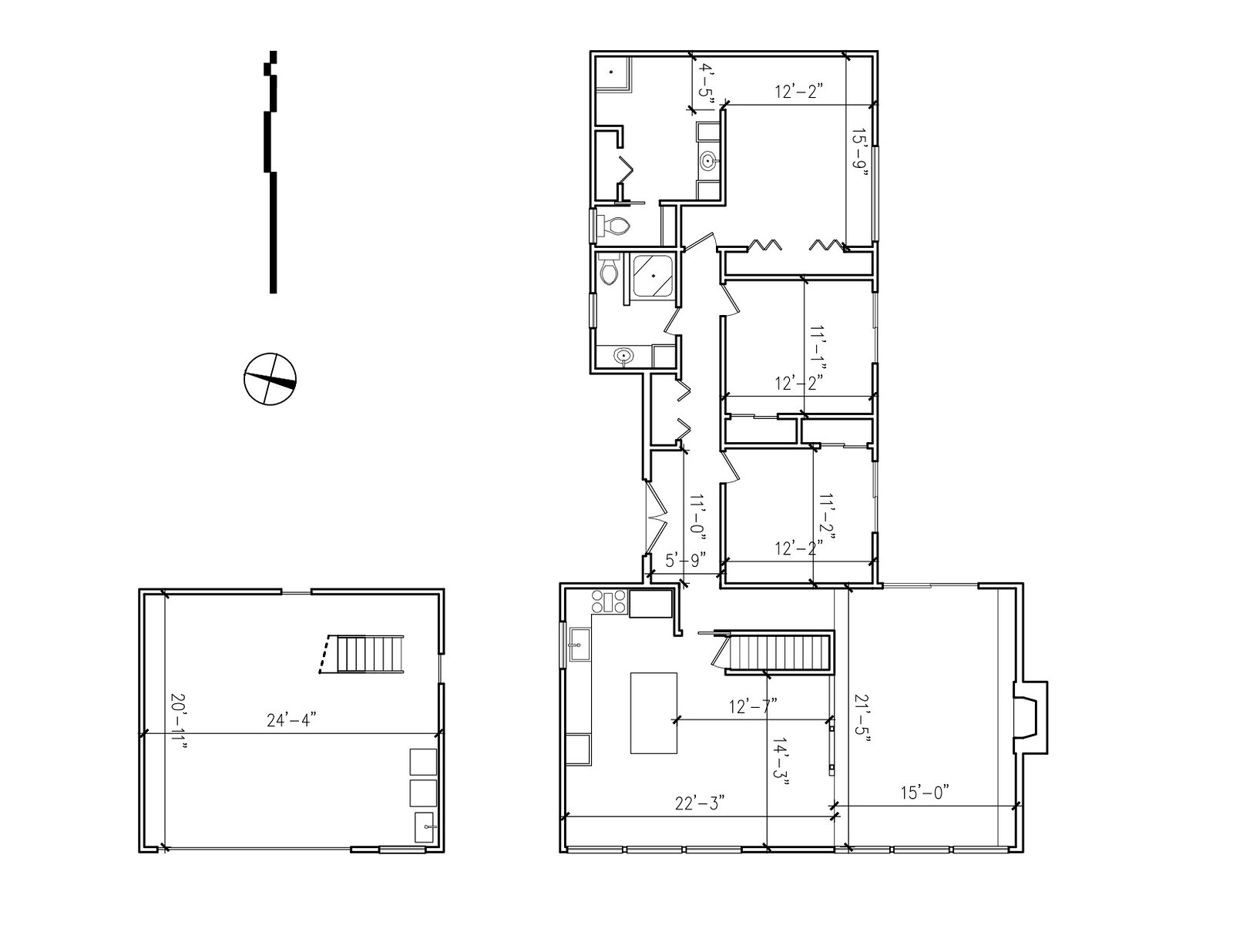This image is a detailed blueprint for a residential layout, potentially a house or apartment. In the bottom left corner, there's an upstairs area measuring 20 feet by 11 feet and 24 feet by 4 inches. A stairway is visible, leading downstairs, and at the bottom right of this room, a sink is positioned.

To the right side of the blueprint, the rest of the residence is illustrated. The entrance is located at the bottom right, leading into a sizable room measuring 21 feet 5 inches in length and 15 feet in width. This room transitions into another area that features a staircase leading upstairs. To the left side of this stairway room is a kitchen, which measures 22 feet 3 inches in width by 14 feet 3 inches in length, with a distance of 12 feet 7 inches from the wall to the island in the kitchen.

A corridor extending 11 feet opens up to a closet that measures 5 feet 9 inches. The layout includes three bedrooms: two of equal size, each measuring 11 feet 2 inches by 12 feet 2 inches, and a larger master bedroom measuring 12 feet 2 inches by 15 feet 9 inches. Adjacent to the master bedroom is a closet of 4 feet 5 inches, leading into the master bathroom. Additionally, there is a second bathroom accessible from the corridor.